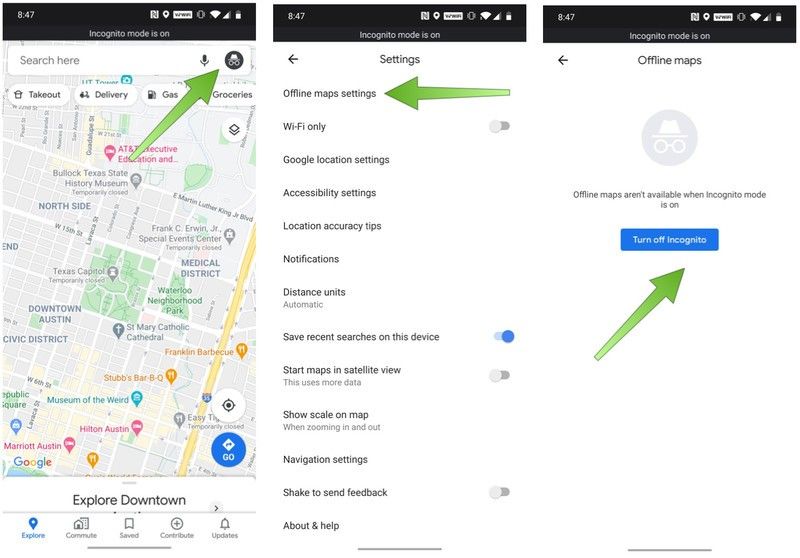The image consists of three mobile screenshots displayed side-by-side from left to right. 

**First Screenshot (Left):** 
The user is in a GPS application, accessed via Google Maps in incognito mode, as indicated by the incognito icon (a fedora with glasses) on the top right corner. The bottom of the screen features five navigation tabs: "Explore," "Commute," "Saved," "Contribute," and "Updates." The "Explore" tab is highlighted in blue. The interface displays the text "Explore downtown" at the bottom, though it is partially cut off. On the top, there's a search bar with the placeholder "Search here," accompanied by a microphone symbol and the incognito icon. Additionally, there are quick access icons for categories like "Takeout," "Delivery," "Gas," "Groceries," and a button for map layers. A green arrow is pointing to the incognito icon.

**Second Screenshot (Middle):** 
The screen shows the settings menu of the GPS application. Various options are listed in a simple white background with black text. A green arrow highlights the option at the top, "Offline maps settings."

**Third Screenshot (Right):** 
This screen focuses on the "Offline maps" section within settings. It prominently displays the incognito logo at the top, followed by a message stating, "Offline maps aren't available when incognito mode is on." Below this message is a large blue button labeled "Turn off incognito," and a green arrow points to this button. 

Capturing the sequence and emphasizing the navigation process within the application, the screenshots highlight the limitations of using offline maps in incognito mode and provide instructions on how to disable incognito mode to access offline maps.